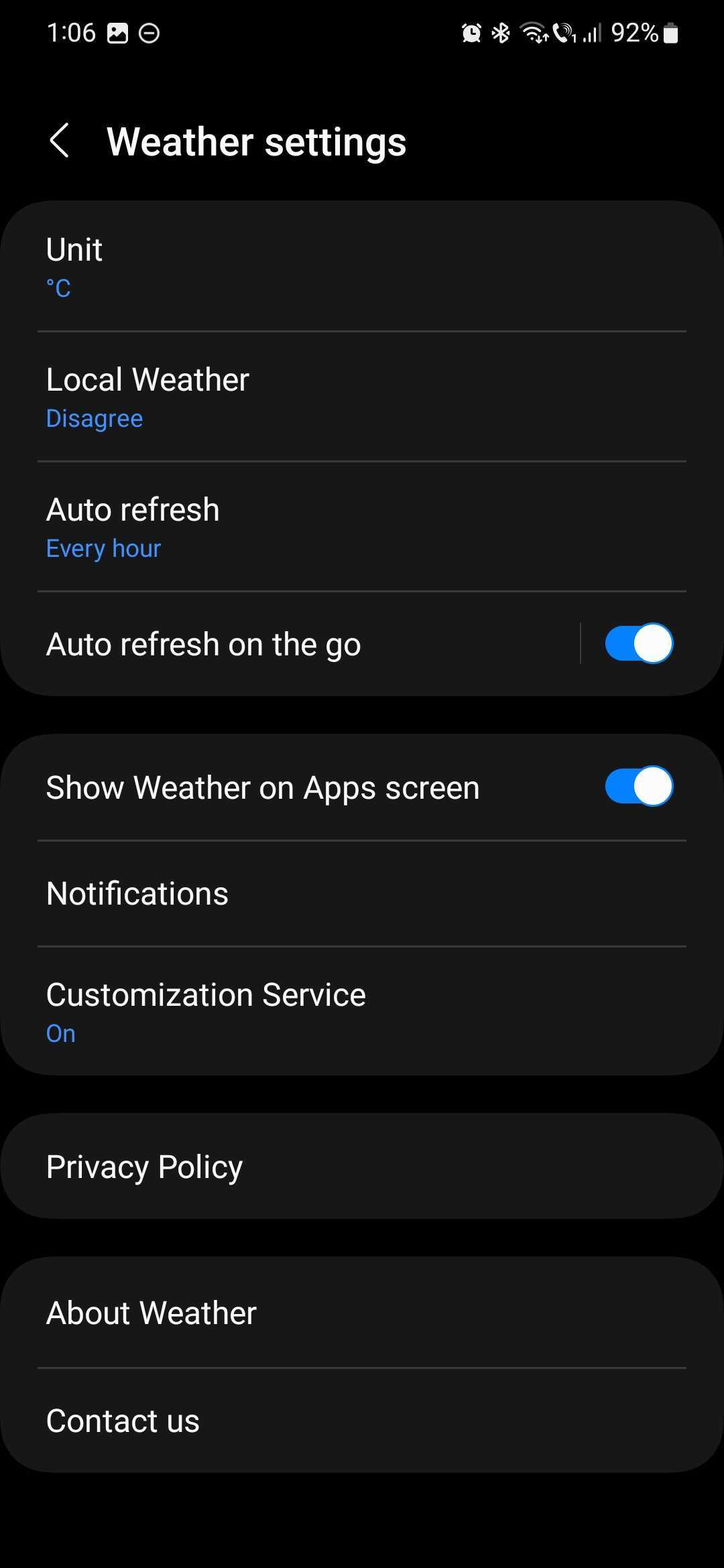The image depicts a detailed view of a smartphone's weather settings screen against a blackish-grey background. At the top, the status bar reveals a few details: the time is 1:06, the battery is at 92%, the Wi-Fi signal is strong, Bluetooth is disabled, and there is an active alarm clock. The settings list several options: 

- "Unit" is highlighted in blue and set to degrees centigrade.
- "Local Weather" is currently set to "disagree."
- "Auto Refresh" is configured to update every hour, and "Auto Refresh on the go" is enabled.
- "Show Weather on App Screens" is enabled.
- The status of "Notifications" is unclear.
- "Customization Service" is turned on.

At the bottom of the screen, there are options for the "Privacy Policy" concerning weather data and a "Contact Us" link. This comprehensive view emphasizes that the user is engaged in customizing their weather settings on their smartphone.